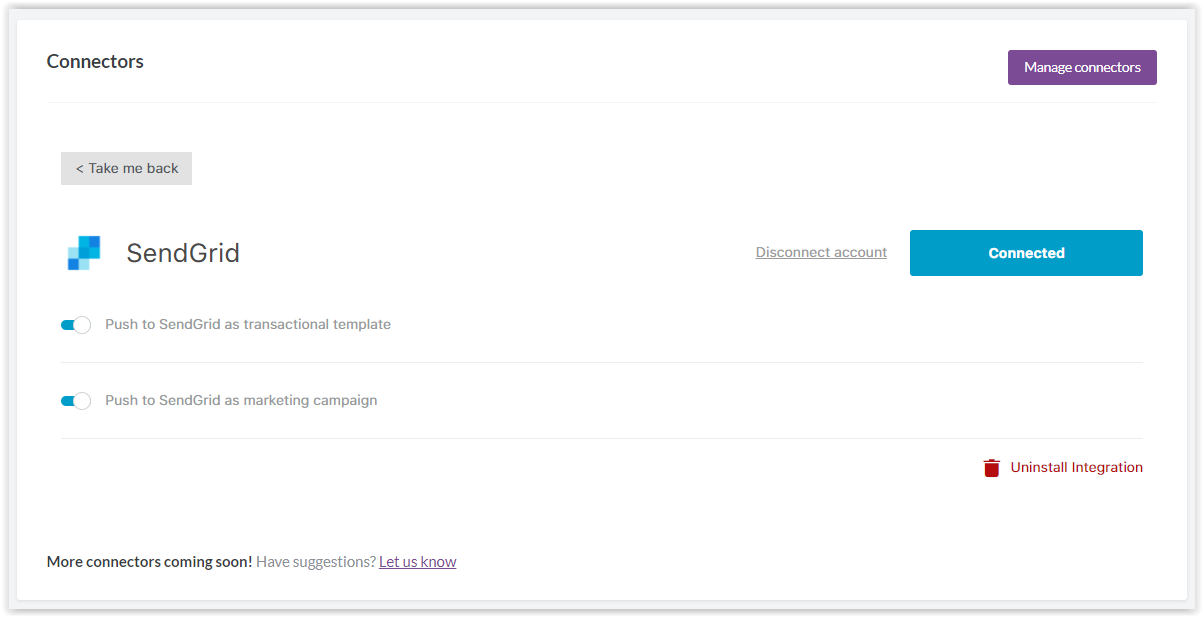Here is a refined and detailed caption for the described image:

---

The screenshot features a white background with predominantly black text and several interactive elements. On the right-hand side, there is a prominent purple button with white text labeled "Manage Connectors". On the left-hand side, the heading "Connectors" is displayed in bold black letters. Below this heading, there is a gray rectangle containing a left-pointing arrow and the text "Take Me Back".

Further down, the screenshot showcases two diagonally stacked blue boxes next to the large black text "Send Grid". Below these boxes, two toggles are visible, both switched to the right. The first toggle states "Push to Send Grid as Transactional Template", and the second toggle reads "Push to Send Grid as Marketing Campaign".

At the bottom of the image, a concluding line reads "More Connectors Coming Soon! Have Suggestions?", followed by a purple hyperlink with the text "Let Us Know". 

On the far right-hand side, a teal rectangle containing white text reads "Connected". Adjacent to this, there is gray text with a hyperlink that says "Disconnect Account".

---

This caption meticulously describes the layout and content of the screenshot, providing a clear and detailed overview.